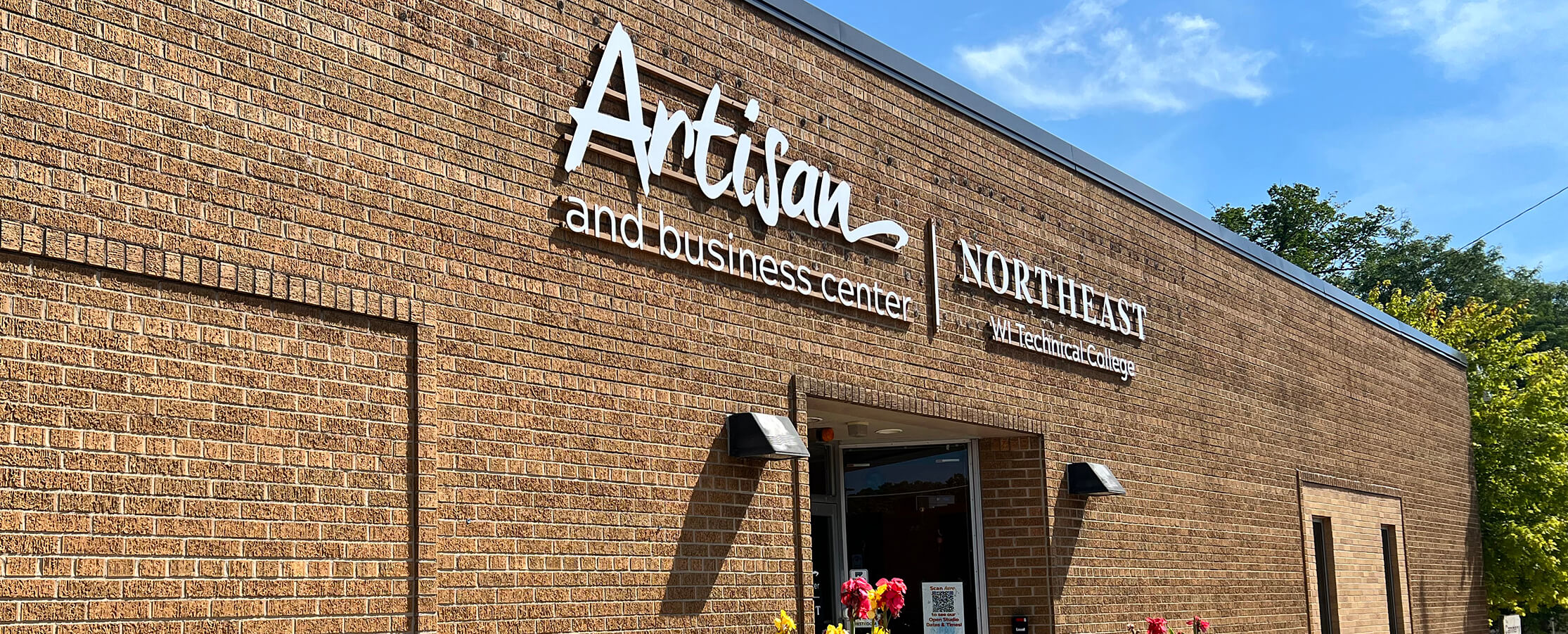This image captures a detailed, close-up view of the entrance to a business building, predominantly showcasing a dark brick facade with a smooth, aluminum gutter in dark blue lining the roof. On the upper part of the wall, centered and white against the dark bricks, large letters spell out "Artisan and Business Center" on the left half of the sign, and "Northeast Technical College" on the right half. Directly beneath this signage is a glass door framed in metal, surrounded by the same dark bricks. A flyer with a QR code is posted on the door, though its exact words are not legible. Adjacent to the entryway are brown light fixtures, one on each side, flanking some visible flower tops poking up in front of the door. Further right in the image, parts of a green tree are seen extending into the frame, overlaid against a backdrop of blue sky with some white clouds.